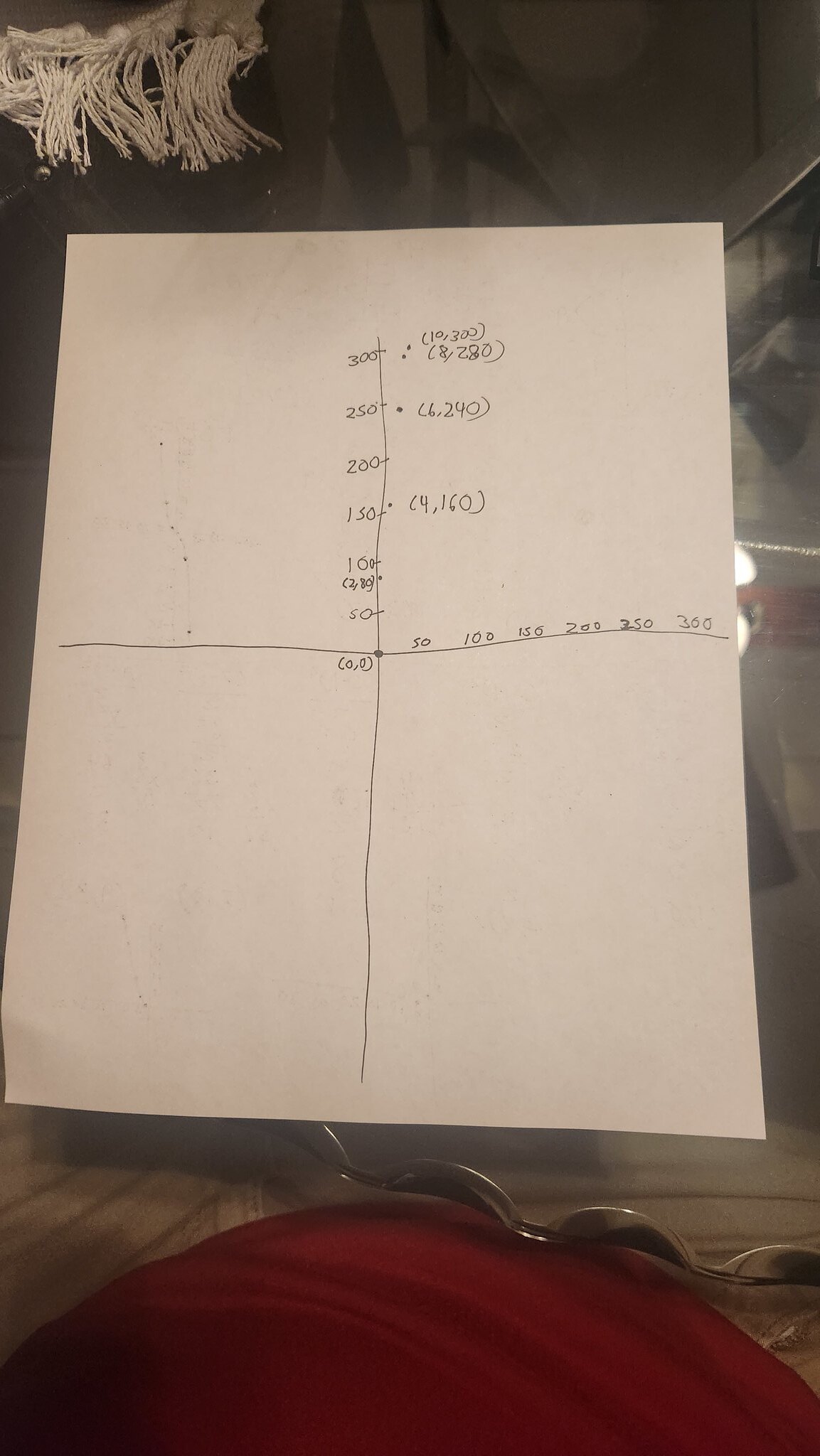The image features an overhead view of an 8.5 x 11-inch sheet of paper placed on a clear glass table. The table itself has a unique texture, featuring silver, wavy patterns that add a sense of dimension and contrast. Surrounding the paper and table surface is an off-white background with tassel-like strings hanging down, resembling mop strings but seemingly attached to a different object. 

On the paper, there is a long horizontal line intersecting with a long vertical line, creating a plus sign with a dot at the intersection. Various numbers are printed along the top edge and the right side of the paper, with additional numeric annotations filling the upper-right quadrant. 

The bottom part of the image shows a rounded, red object with varying shades of red, including darker and lighter areas, possibly due to shadows being cast upon it. The photograph captures subtle details such as shadows and smudges on the paper, contributing to a realistic and intricate depiction.